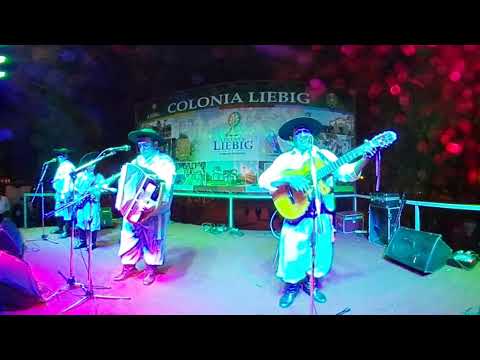This vivid photographic image captures an energetic Hispanic band performing on stage, likely indoors. The focal point is a man resembling a cowboy or gaucho, standing left of center, holding an electric guitar and singing into a microphone. He dons a white hat, baggy pants, an oversized shirt, black boots, and a bandana mask across his face. Beside him, another man clad in similar attire plays an accordion. In the background, two other men are visible; one, without an instrument, seems to be singing into a microphone, while the fourth member stands passively, possibly by a xylophone. The stage is set against a colorful backdrop featuring a sign that prominently displays "Colonia Liebig" twice, accompanied by graphics of buildings and a sphere. The scene is lit with a combination of white, purple, red, blue, and green strobe lights, with the most prominent musician bathed in a mix of white and bluish light against a predominantly red-lit background. Black horizontal bands frame the top and bottom of the image, adding to its dynamic composition.